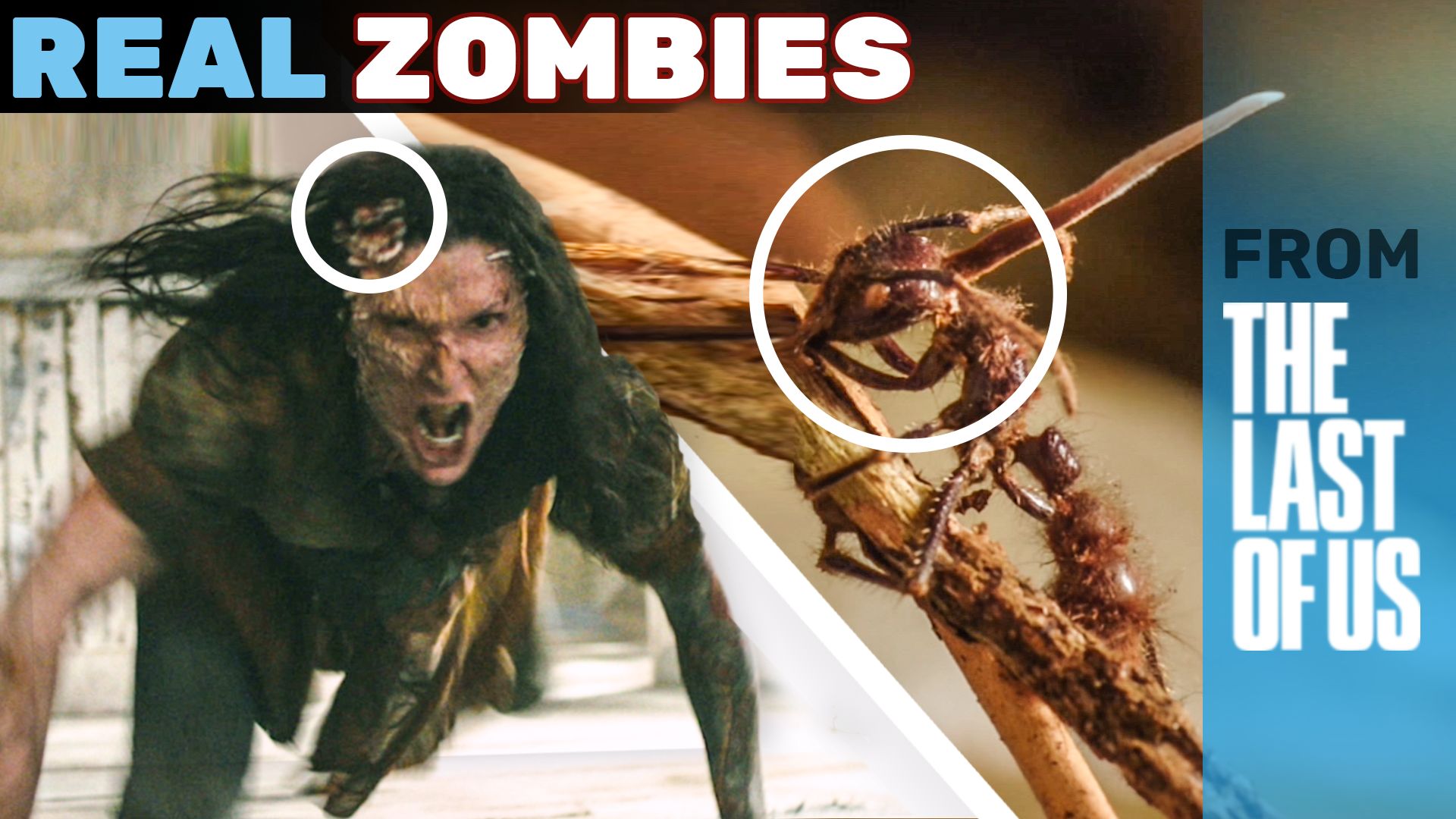In this horizontal landscape photographic image set outdoors, resembling a movie or TV show advertisement, a white man is captured racing towards the camera in an aggressive pose, his mouth open in anger. Dressed in dark clothes and having distinctive features including long dark hair and substantial black hair on his left arm, his face appears adorned with hanging skin to create a fearsome look akin to that of a zombie. Situated prominently on the upper left, the sign reads "Real Zombies" with 'Real' in blue and 'Zombies' in white, emblazoned on a black border. A vertical gradient blue border on the right contains the white text "The Last of Us" and a line of black text reading "From." Notably, a white circle highlights a close-up image of an ant on a gray branch to the right side of the photograph, further implying a connection to the theme of a brain-eating creature, possibly representing the transformation depicted in "The Last of Us" series. The composition and elements collectively convey an intense, immersive experience into a world affected by a zombie apocalypse.